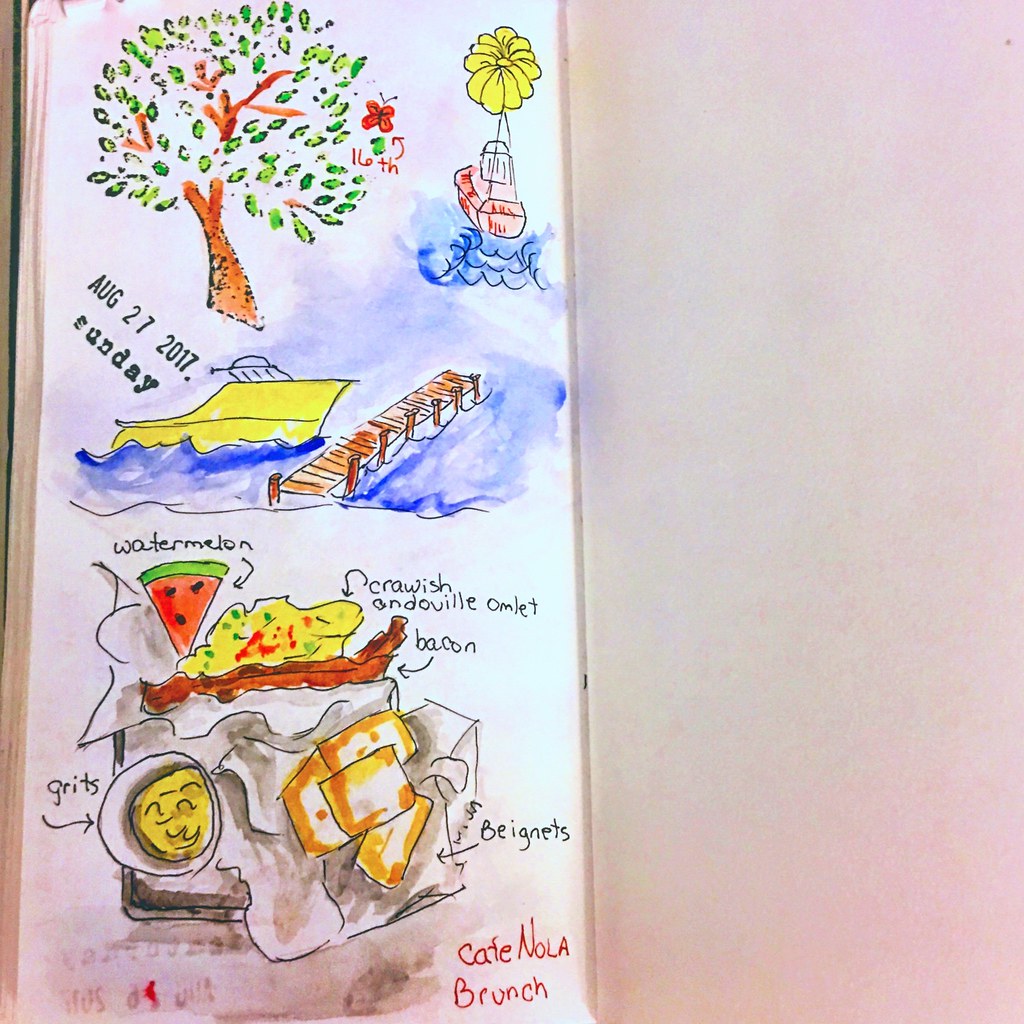The image features a detailed, painted menu displayed on a narrow, white surface to the right. The vertical surface is contrasted by a gray background on the left, and a faint green vertical stripe with a wooden tone can be glimpsed at its far left edge. The painting itself showcases various colorful elements including a brown and green tree, a yellow flower, a white and red boat, and blue water. Another segment depicts a yellow boat docked near a brown pier, all set against the water.

Additional visuals include a slice of watermelon and another image potentially depicting a yellow and brown boat, with another yellow object beneath it. Each visual element is accompanied by black-lettered labels with arrows indicating "Beignets," "Bacon," "Crawfish," an unidentifiable word, "Omelet," "Watermelon," and "Grits." The bottom right corner features the text "Kate Nola Brunch" in bright red letters. Additionally, a date stamp at the bottom reads "8-27-2017, Sunday."